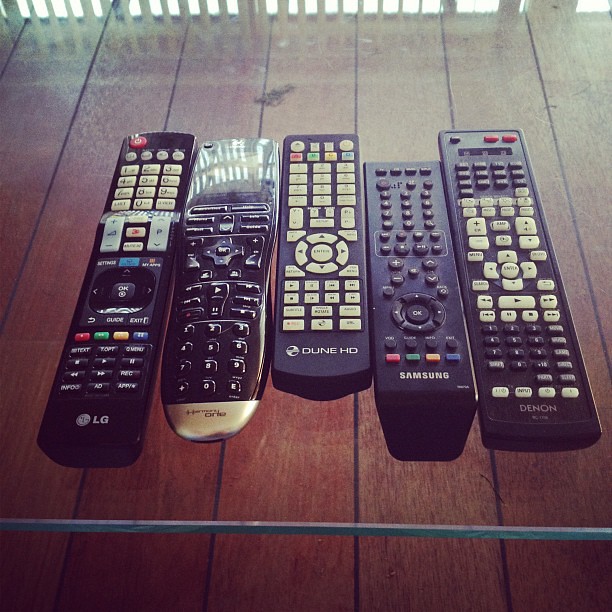The image is a detailed overhead photograph of five devices, primarily remote controls, on a glass-topped dark brown wooden surface with darker brown to black stripes. Four of the devices are distinct remote controls, and one resembles a phone but likely is also a remote given the small square screen at the top. All remotes are predominantly black. 

The brands are identifiable: LG, Samsung, Dune HD, and Denon. One remote says Harmony One. Button layouts vary across the devices — one remote features exclusively black buttons, another combines white and black buttons, and two remotes have all white buttons. The LG remote includes colorful buttons in red, green, yellow, and blue. The Samsung remote, noted for a mix of black and white buttons, also features four colored rectangular buttons. The devices rest on what appears to be a glass surface through which the patterned wood beneath is visible. 

This photograph aptly showcases the variety and design of the remote controls, highlighting their commonality in color but diversity in brand and button configuration.